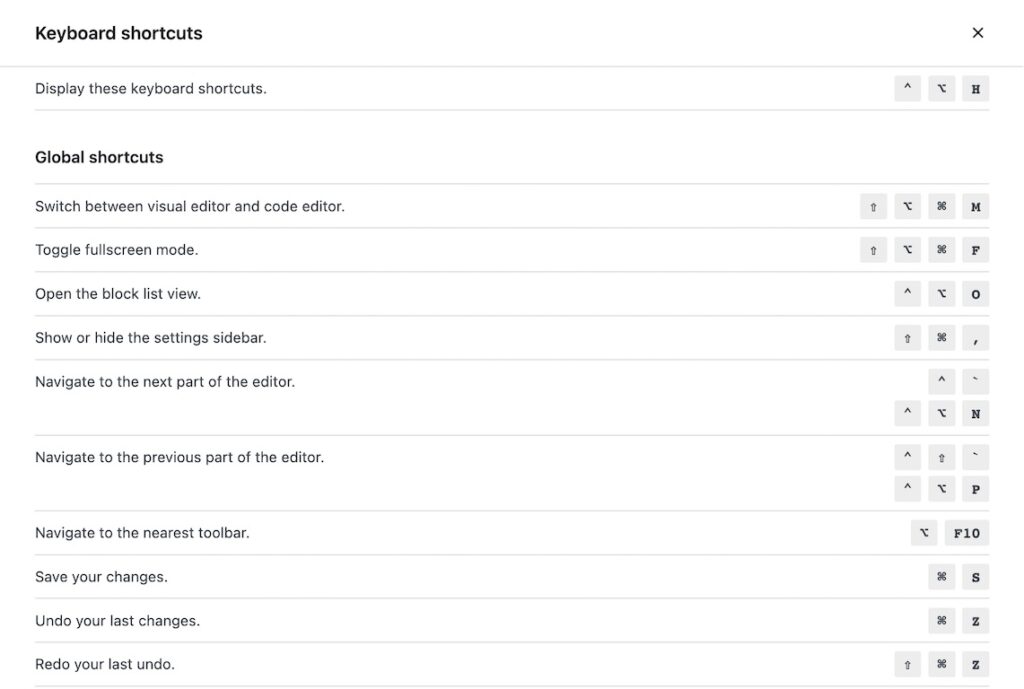This is a detailed screenshot of a website page listing numerous keyboard shortcuts for various actions. At the top, there is a section labeled "Display These Keyboard Shortcuts," accompanied by small gray squares representing the corresponding key combinations. Below this, the shortcuts are categorized under "Global Shortcuts."

Each global shortcut is listed with a description followed by the key combination necessary to execute it. Notable shortcuts include:

- "Switch between Visual Editor and Code Editor"
- "Toggle Full Screen Mode"
- "Open the Block List View"
- "Show or Hide the Settings Sidebar"
- "Navigate to the Next Part of the Editor"
- "Navigate to the Previous Part of the Editor"
- "Navigate to the Nearest Toolbar"
- "Save Your Changes"
- "Undo Your Last Changes"
- "Redo Your Last Undo"

Each key combination is displayed in a small gray square, mimicking the appearance of the actual keys on a keyboard. The overall design features a white background with the shortcuts listed in black font, providing clear and easy-to-read instructions for users. This organized layout allows for efficient navigation and utilization of keyboard shortcuts.